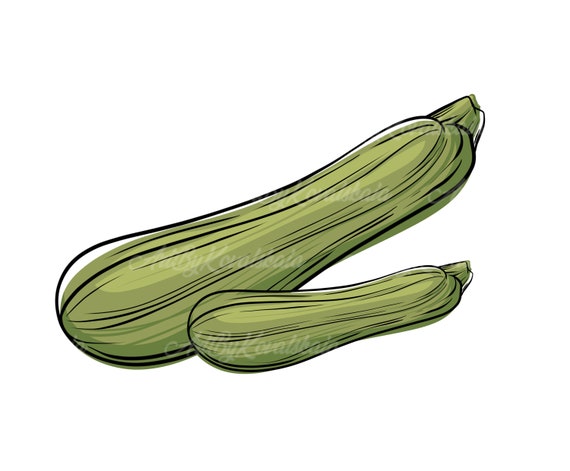The image is a hand-drawn, or possibly digitized, illustration of two green zucchinis. The larger zucchini is prominently positioned at the top and is slightly slanted upwards, with its stem pointing to the right. The smaller zucchini is positioned below the larger one, also oriented with its stem to the right but is less slanted. Both zucchinis are primarily green with black streaks and lines detailing their texture and shape. The scene includes a mix of black, white, green, and lighter green colors. There is some text in white on the image, but it is too faint to be legible. The style of the illustration suggests watercolor or digital art, capturing the simple, yet intricate, appearance of the zucchinis.